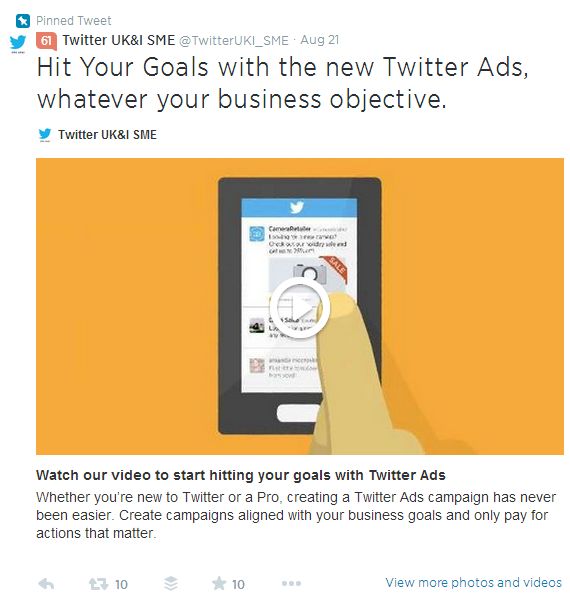The image displays a Twitter advertisement page. At the top, there is a "Pinned Tweet" label accompanied by an icon of a white pin against a blue background. The account "Twitter UK & SME" is identifiable by its blue bird logo and its handle, @TwitterUK_SME, dated August 2021. 

The pinned tweet reads: "Hit your goal with the new Twitter ads, whatever your business objective." Below this, there's an embedded video, indicated by a white play button. The still from the video features a brown-skinned hand pointing to or touching a smartphone. The smartphone, which has black bezels, is showing the Twitter app on its screen. The background of the video is a solid orange color.

Beneath the video, there's black text: "Watch our video to start hitting your goals with Twitter ads. Whether you are new to Twitter or a pro, creating a Twitter ad campaign has never been easier. Create campaigns aligned with your business goals and only pay for actions that matter."

At the bottom of the tweet, typical Twitter interaction buttons appear: a back button, a retweet button showing 10 retweets, and a like button showing 10 likes. On the bottom right, there is a "View more photos and videos" link in blue.